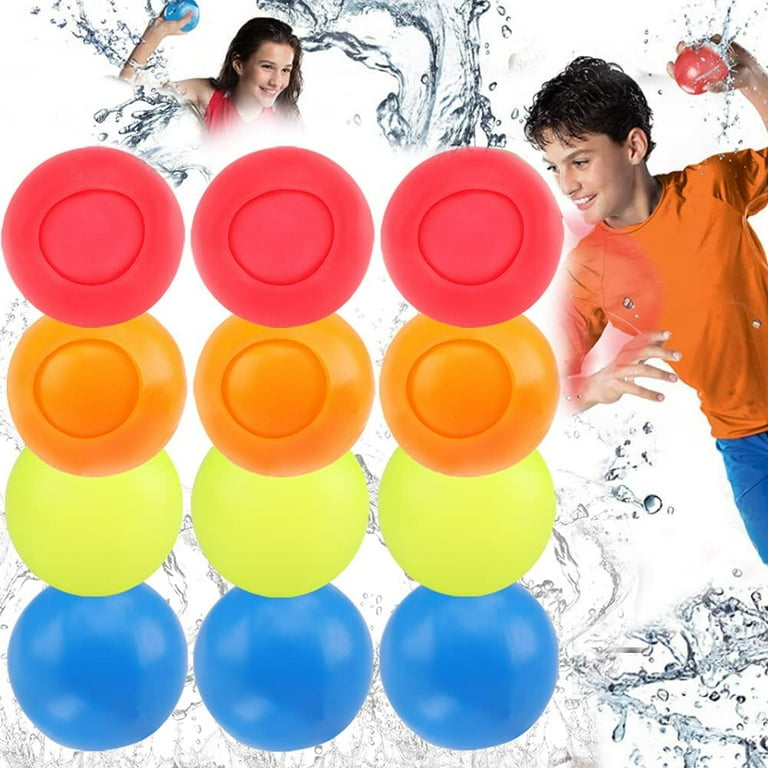The image is a colorful advertisement showcasing a fun children’s toy designed for water play. In the background, there are splashes of water, creating an energetic and playful atmosphere. At the center of the image, prominently displayed, are 12 sponge balls, arranged in four rows of three. The top row is pink, the second row is orange, the third row is yellow, and the bottom row is blue, indicating a variety of vibrant colors.

On the left side of the image, a girl with long black hair and a bright smile is visible. She is wearing a red sleeveless shirt and holding a blue sponge ball in her right hand, poised to throw. To the right, a boy with short dark hair, clad in an orange shirt and blue shorts, is also grinning happily. He is holding a red sponge ball in his left hand, appearing ready to launch it. His ball shows water spraying out, emphasizing the water-absorbing and spraying feature of the toys. Together, the children’s joyful expressions and dynamic poses convey the excitement and playful potential of the sponge balls.